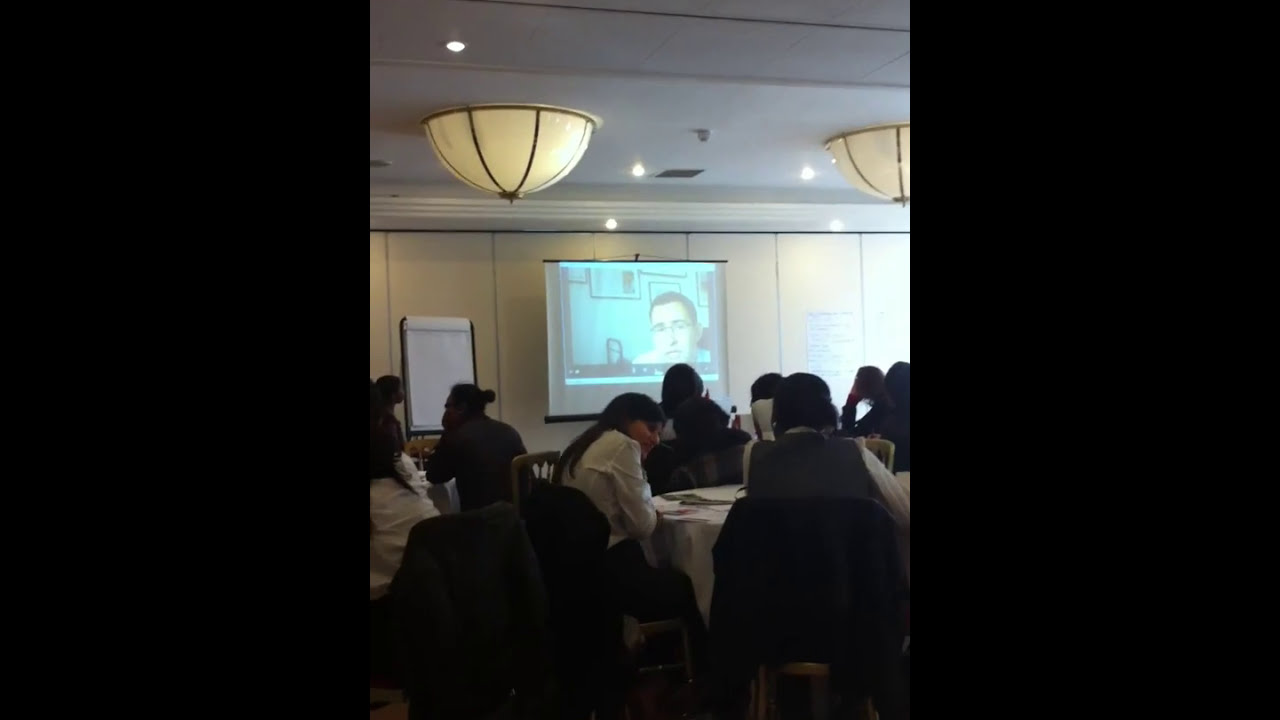This photograph captures a bustling meeting room filled with an engaged audience of both men and women, seated at round tables draped with white tablecloths. Attendees are absorbed in the presentation on a projector screen, where a man with glasses and short hair, possibly the instructor, appears to be speaking. In the foreground, a man in a gray vest with a coat draped over his chair and a woman with long hair wearing a white shirt and dark pants are prominent. To the left of the screen, an easel holds sheets of paper, likely for brainstorming or note-taking. The room's ambiance is well-lit, featuring a mix of large dome lights and smaller fixtures on the white ceiling, with some natural light filtering in from the right side. The walls blend white and wood panels, adding a touch of warmth. Scattered jackets on chairs underscore the formal yet casual atmosphere of the gathering.